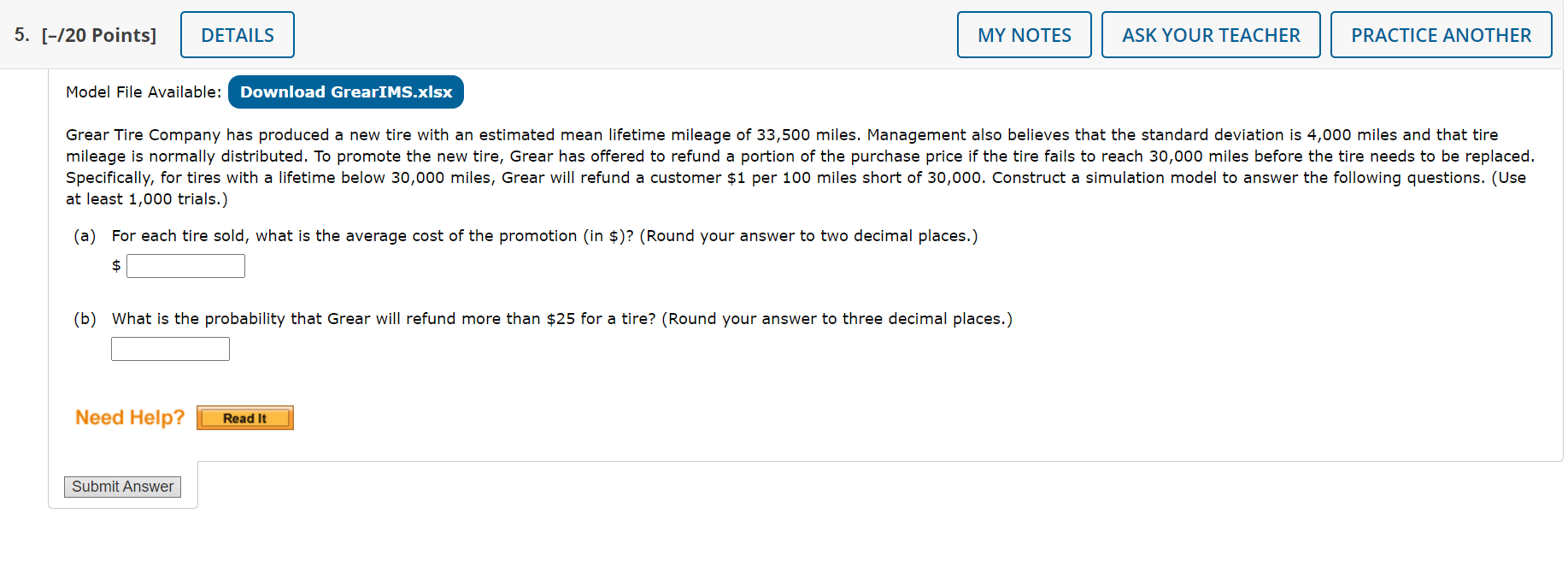A horizontal rectangular image primarily features a white background. At the very top of the image, there's a light blue to light gray gradient banner. On the far left of this banner, the text "5.5. [ -/20 points ] Details" is displayed within a light gray box with a blue border. Adjacent to this box are three additional rectangular gray boxes with blue borders labeled "My Notes," "Ask Your Teacher," and "Practice Another."

Below these boxes, in small black letters, there's text that reads "Model file available:". Directly beneath, there's a dark navy blue button with gray text labeled "Download GreerIMS.xlsx."

Following this button is a paragraph in tiny black text which reads: "Greer Tire Company has produced a new tire with an estimated mean lifetime mileage of 33,500 miles. Management also believes that the standard deviation is 4,000 miles and that tire mileage is normally distributed. To promote the new tire, Greer has offered to refund a portion of the purchase price if the tire fails to reach 30,000 miles before the tire needs to be replaced. Specifically, for tires with a lifetime below 30,000 miles, Greer will refund a customer $1 per 100 miles short of 30,000. Construct a simulation model to answer the following questions. (Use at least 1,000 trials.)"

Beneath this paragraph are two questions labeled A and B that need to be answered, followed by a gray box intended for submitting the answers. On the right side, there's an orange "Need Help?" label next to an orange button.